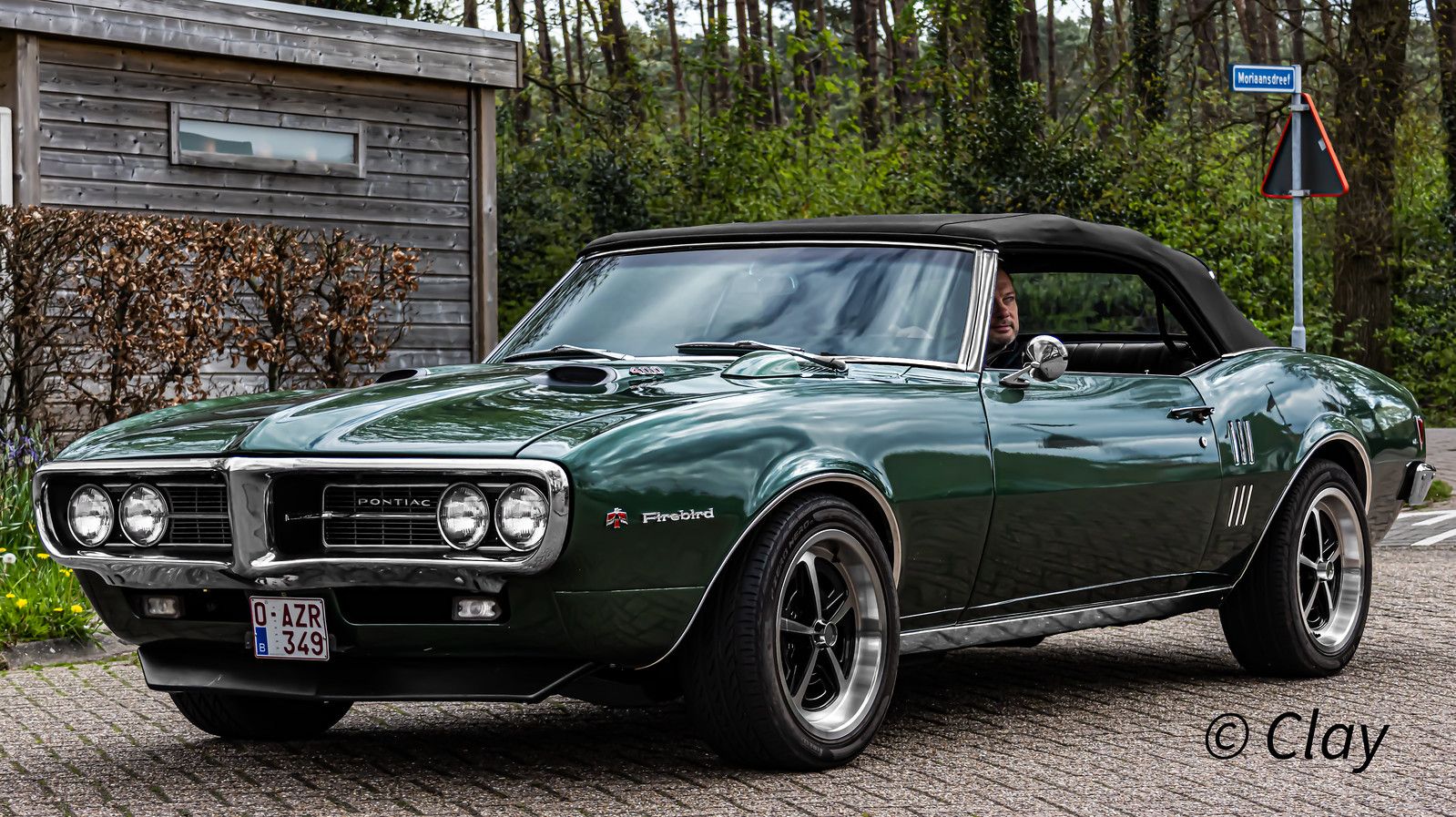In this outdoor image, a fully restored, dark hunter green Pontiac Firebird convertible from the 1960s sits prominently on a brick-paved road. Its bright chrome trim gleams in the natural light, accentuating the classic design of the vehicle. A Caucasian man with a black mustache and wearing a black shirt is seated in the driver’s seat, gazing out of the window.

The scene is set in a European country, as indicated by the license plate number 0AZR349. The background features a weathered wooden building with dead bushes in front and a lush stretch of greenery further back, contributing to the rustic charm of the setting. Additionally, a street sign is partially visible at the corner, suggesting the car is parked near an intersection. The bottom right-hand corner of the image bears a copyright note, "Clay."